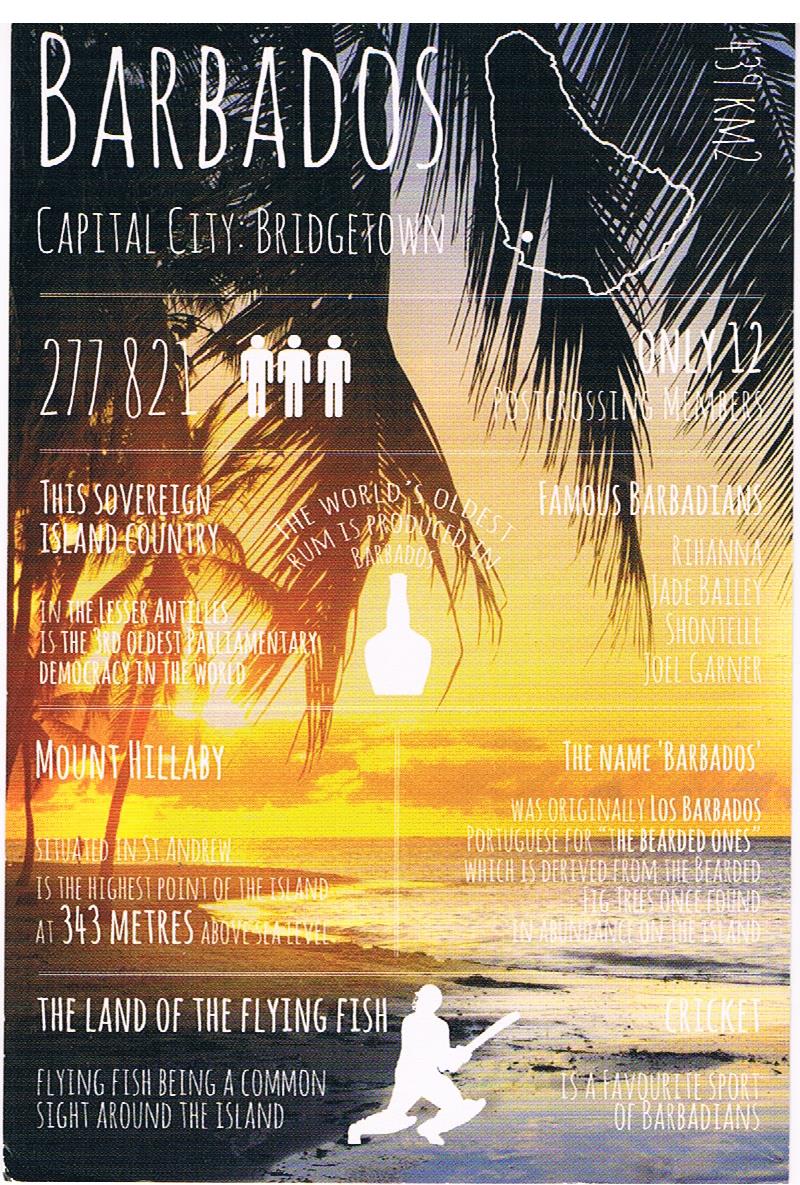The poster for Barbados features an idyllic beach scene with gray sand on the left and shimmering water on the right, transitioning to a warm orange hue as it meets the horizon under an orange sky dotted with clouds. Palm tree fronds hang down from the top, setting a tropical ambiance.

Centered at the top of the poster, bold text reads "Barbados, Capital City, Bridgetown," accompanied by a white outline of the island. This is followed by various rectangular sections of text separated by thin white lines. The banner displays the population figure of "277, 821" and highlights that Barbados is a "Sovereign Island Country" with Bridgetown as its capital. 

Prominent facts about Barbados are presented, including its standing as the third oldest parliamentary democracy in the world and being home to the world's oldest rum. Famous Barbadians such as Rihanna, Jade Bailey, Shantelli, and Joel Garner are listed. 

The poster also notes that "Mount Hillaby situated in St. Andrew is the highest point of the island at 343 meters above sea level" and explains that the name Barbados comes from "Los Barbados," Portuguese for "the bearded ones," referencing the once plentiful bearded fig trees. 

The lower section of the poster champions Barbados as "The land of the flying fish," noting these fish are a common sight around the island. Additionally, it mentions the popularity of cricket in Barbados, with the image of what may be a cricket player enhancing this point. Overall, the poster combines vibrant imagery with in-depth facts, enticing viewers to explore the rich history and culture of Barbados.